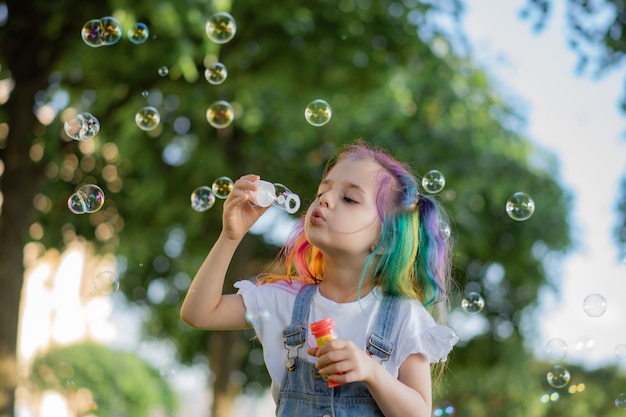The image features a young Caucasian girl, approximately 7 to 8 years old, with vibrant rainbow-colored hair showcasing shades of green, yellow, purple, blue, and reddish-orange. She is engrossed in the act of blowing bubbles, holding a bubble dispenser in her left hand while using an applicator to create bubbles with her right hand. She is dressed in a white t-shirt with frayed armholes, layered under blue denim overalls. The focal point captures her mid-blow, her eyes fixated on the bubble wand, unaware of her surroundings. Numerous bubbles of varying sizes float around her. The background, which is blurred out, appears to be a park or a garden with visible greenery and a tree, suggesting it is daytime.